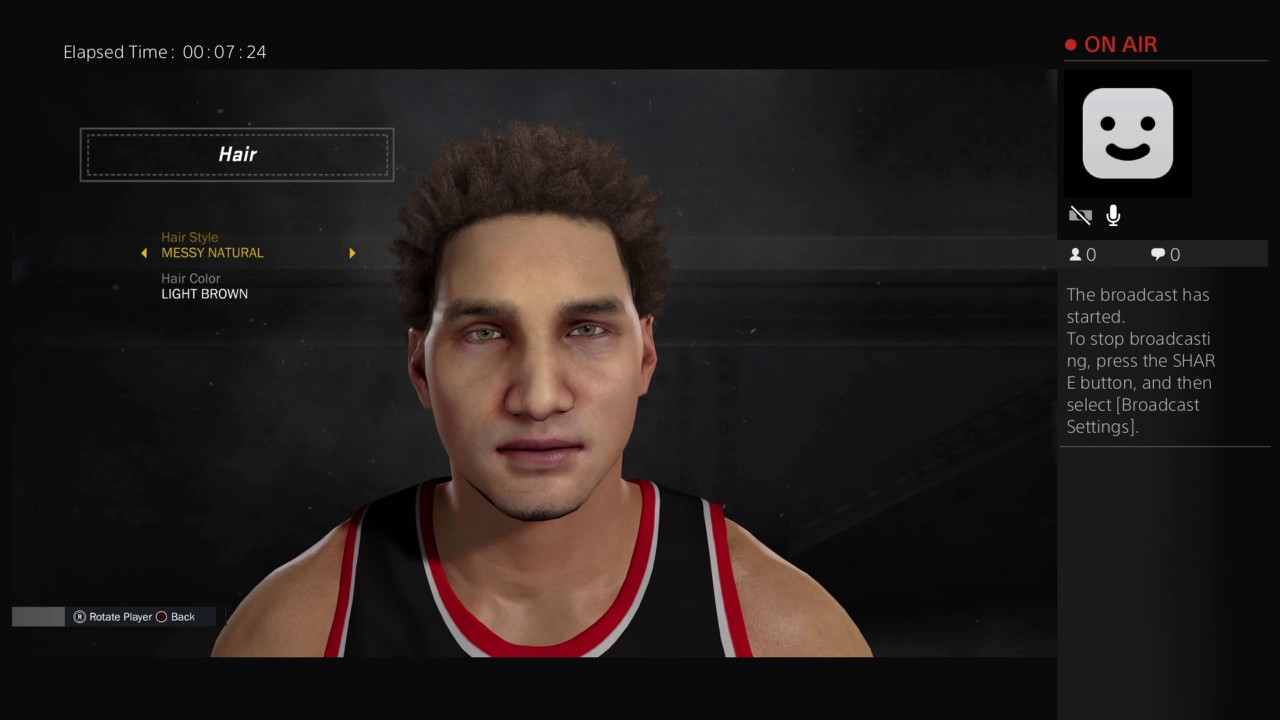The image is a screenshot from a hyper-realistic video game interface, predominantly black in background. At the top center of the screen, the elapsed time reads "00:07:24". To the right, the words "On Air" are displayed in red font accompanied by a red circle, indicating a live broadcast. The foreground showcases a character customization menu where the player is selecting the appearance of their basketball player avatar. The customization options are highlighted, specifically on 'Hair Style' labeled as "Messy Natural" and 'Hair Color' as "Light Brown". The avatar, a basketball player, has short light brown hair and light-colored eyes. They are dressed in a black jersey with white and red accents. Instructions at the bottom prompt the user to "Rotate Player" or use the "Back" button. To the right, there is a small square icon featuring a smiley face, suggesting the camera is off but the microphone is active.